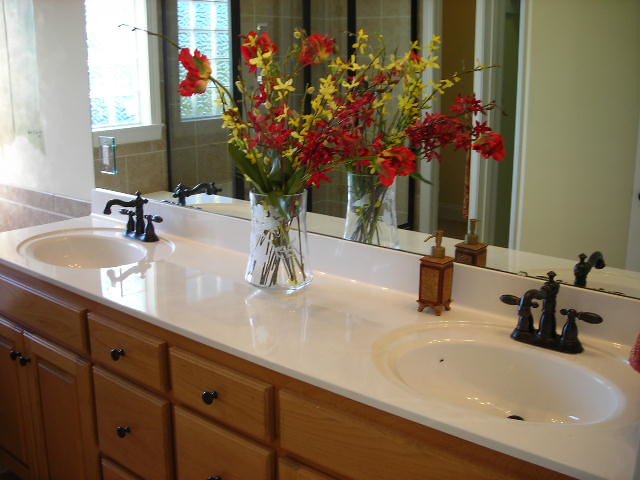The photograph, taken indoors during daytime, showcases a section of a bathroom focusing on the double sink area. The composition highlights a pair of oval sinks set into a glossy, white counter that stretches along the breadth of the image. Each sink is equipped with elegant, black, wrought iron faucets and handles. The sinks are noticeably spaced apart, enhancing the room's sense of space and luxury.

To the left of the right sink stands a distinctive brown soap dispenser, elevated on four small, brown legs, adding a touch of rustic charm to the modern setup. Centrally positioned between the two sinks is a large white vase adorned with subtle etchings, filled with a vivid arrangement of red and yellow flowers. The yellow blooms appear to be forsythias, their stems clearly visible through the transparent vase, adding a splash of natural color and elegance to the scene.

The background features an expansive mirror, reflecting and amplifying the light and spaciousness of the bathroom. Below the counter, the storage areas consist of brown drawers and cabinets, each fitted with small, round, dark knobs that provide a classic contrast to the contemporary sink and counter design. On the right side of the image, the mirror captures the reflection of a sunlit window, allowing natural light to filter into the room and enhancing the overall warmth and inviting atmosphere of the bathroom.